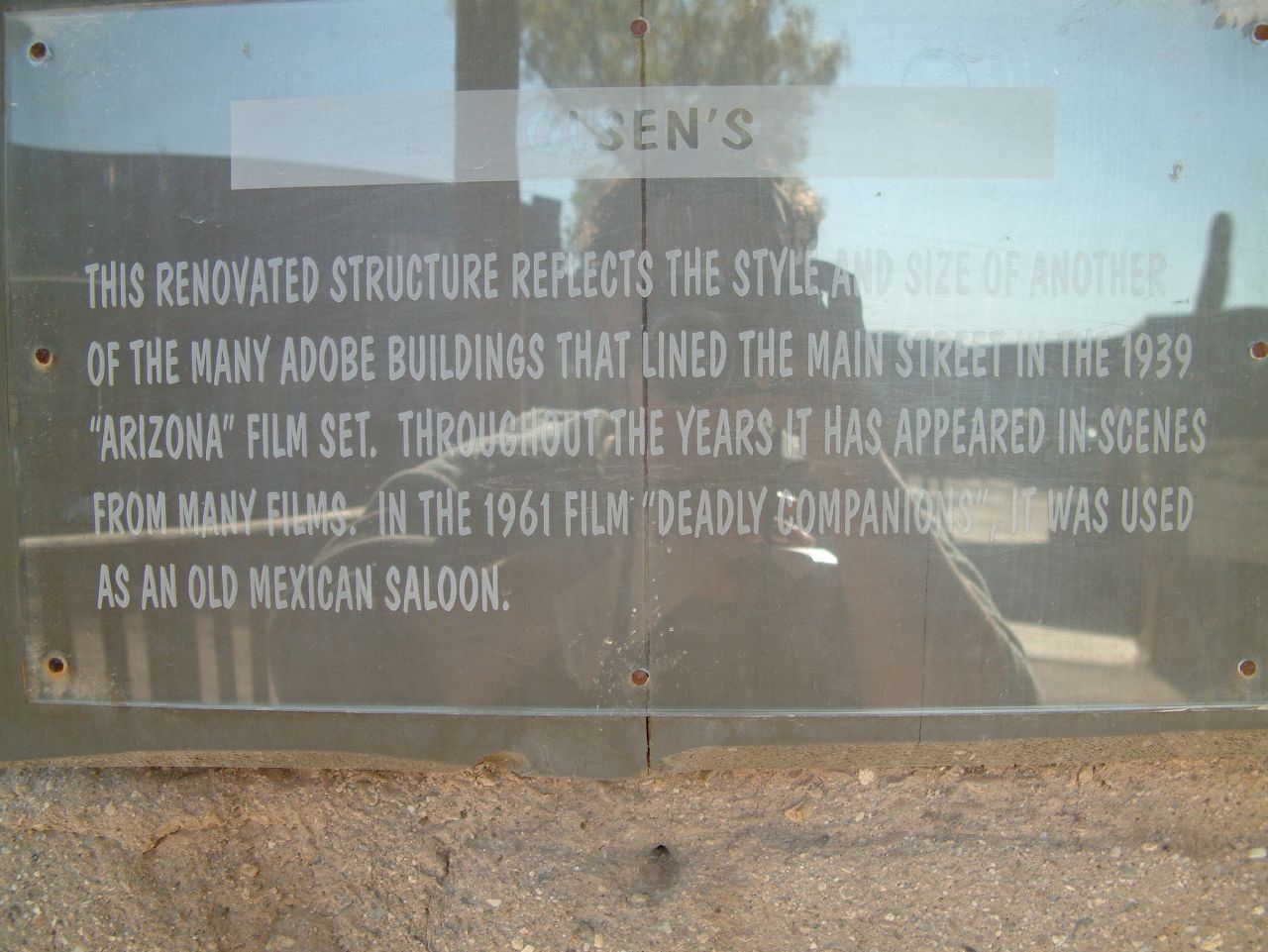The image is a color photograph, in landscape orientation, featuring a reflective, translucent placard mounted on a tan stucco wall. The placard, attached with several rusty screws, provides historical information about the building it adorns. It reads: "This renovated structure reflects the style and size of another of the many adobe buildings that lined the main street in the 1939 'Arizona' film set. Throughout the years, it has appeared in scenes from many films. In the 1961 film 'Deadly Companions,' it was used as an old Mexican saloon." The top panel of the placard, tinted and partially obscured by reflections, appears to bear the title "SEN'S." The photograph captures the entire scene, reflecting the image of the photographer within the glass-like surface of the placard, creating a visual blend with the rocky and dirt ground below, evoking a sense of the historic cowboy film sets.